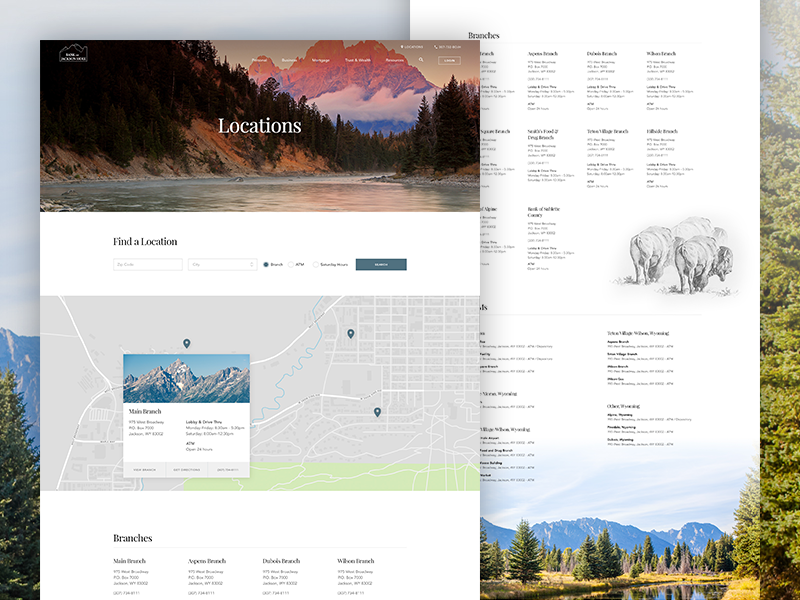**Screenshot of Locations Page**

The image is a detailed screenshot of a web page titled “Locations.” The main page takes the forefront, resembling an open magazine with several layers of pages visible behind it. On the left side, there's a partially obscured landscape picture. On the right, a page loaded with information displays the rear view of three buffaloes with scenic surroundings in the background.

The primary page “Locations” features a large, picturesque banner depicting a sunset over greenish water flanked by what appear to be pine or evergreen trees. Centrally located in white text is the word "Locations." Below the banner, on a white bar, are the words "Find a Location," accompanied by several input fields and a prominent green button on the right side.

Further down, the page transitions to a map view primarily showcasing a grayscale layout of a city with white roads. Three pinpoint markers or bubbles indicate specific locations. A particular bubble highlights a mountain, accompanied by a pop-up. Below this map view is a green bar. Lastly, the bottom section titled "Branches" lists four distinct statements about various branch locations.